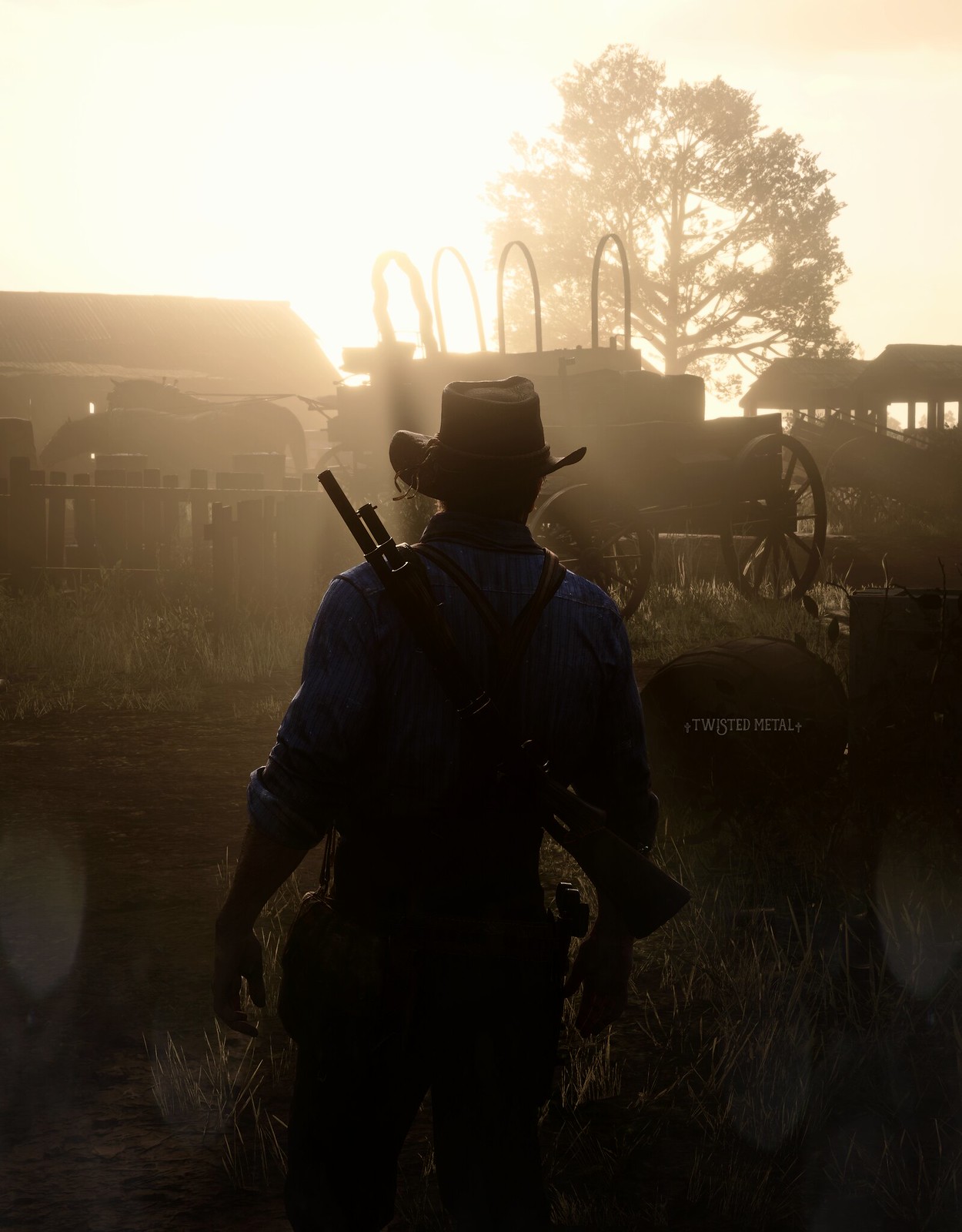A rugged cowboy stands prominently in the foreground of this evocative, western-themed image. Clad in a dirt-streaked, long-sleeved collared shirt with the sleeves rolled up to his elbows, he embodies the essence of a seasoned frontiersman. A rifle is securely strapped to his back, while a gun belt snugly wraps around his waist, housing a pistol ready for a quick draw. His attire is completed by a classic cowboy hat and sturdy suspenders, enhancing his imposing figure.

The setting sun casts a blinding light, creating a striking contrast that darkens the background and adds a dramatic flair to the scene. Behind him, an old-fashioned wooden wagon stands as a testament to bygone days, surrounded by several horses grazing nearby. Accompanying the wagon are wine barrels, one upright and another toppled on its side, emblazoned with the words "Twisted Metal."

The landscape extends with a dirt road cutting through a patch of tall, hay-like grass leading to a humble barn and a solitary tree. The interplay of light and shadow, intensified by the blinding sun, lends a nostalgic and almost surreal quality to the image, evoking memories of the untamed West.